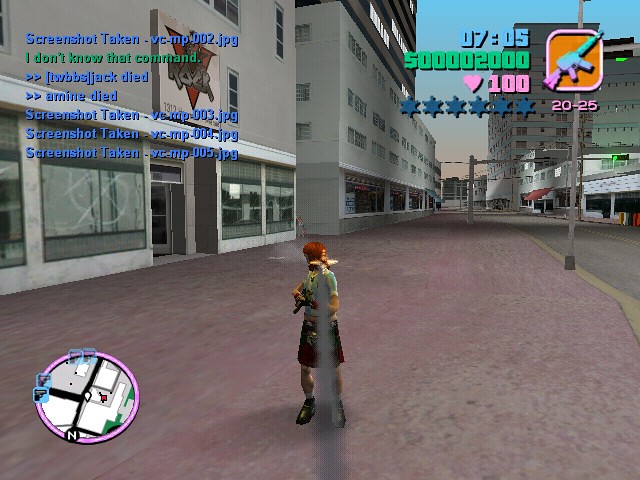This screenshot appears to be taken from the multiplayer component of Grand Theft Auto: Vice City, featuring an array of in-game elements. In the center of the image, a character presumed to be a woman is positioned on a reddish-pink sidewalk, wearing a red skirt and blue top with a weapon aimed toward the viewer. The environment includes gray high-rise buildings, many with signs, windows, storefronts, and graffiti. An ominous atmosphere is depicted with closed or vacant properties. 

In the upper right corner, there's an automatic rifle icon alongside numbers "20-25." Six blue stars are visible, indicating a high wanted level, next to the time "07:05." Below this, a cluster of numbers "5000020000" can be seen, possibly representing in-game stats or a monetary value. 

A gray streak, perhaps due to a screen glitch, runs down the image, affecting visibility. Midway down the left side, a pink circle appears around a minimap or compass, typically showing avatar positioning. The bottom of the image highlights repeated "Screenshot taken" messages with file names like "VCMP002.JPG" and additional phrases such as "I don't know that command" in green and "mind died" in blue. 

Overall, this detailed snapshot provides an eerie vista of Grand Theft Auto Vice City's in-game experience, filled with complex visual and textual elements.